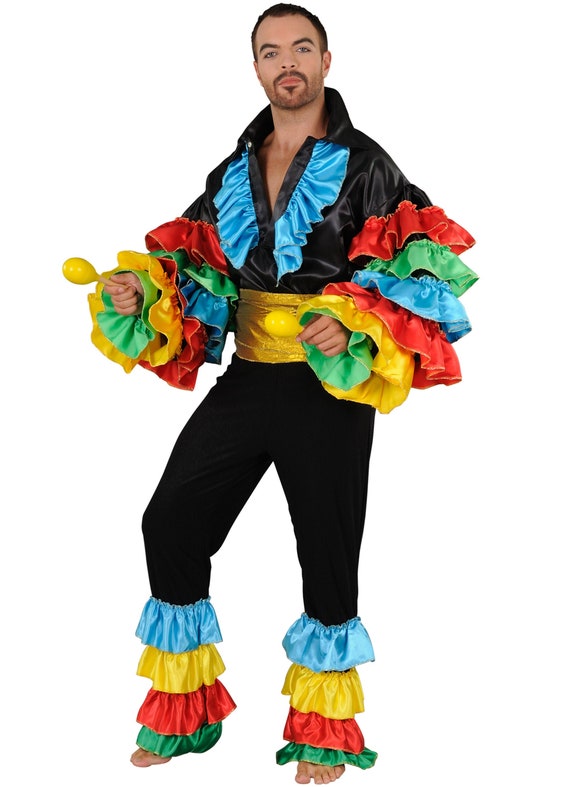This photograph captures a man dressed in an elaborate Latin American dance costume, characterized by intricate multicolored ruffles and distinct ornamental details. He has brown hair, a closely cut beard with a goatee, and a long, round mustache. His outfit consists of a black silk top with a deep V-neck adorned with blue ruffles. The sleeves of his shirt are heavily decorated with large ruffles in a sequence of red, green, blue, red, yellow, and green extending down to his wrists. 

Around his waist, he wears a wide yellow sash, and his black pants also feature similar multicolored ruffles at the cuffs in tones of blue, yellow, red, and green. The man is barefoot, accentuating the vibrant ruffles that continue up from his ankles. As a finishing touch to his costume, he holds a yellow maraca in his hand, further emphasizing his role as a Latin American dancer, potentially in a vibrant performance such as a cha-cha. This detailed ensemble captures the essence and exuberance of traditional Latin American dance attire.